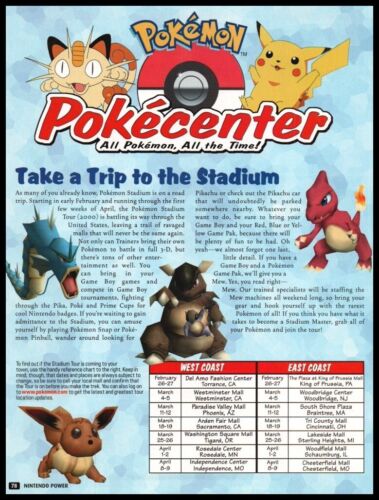The poster titled "Pokemon Pokey Center" features various vibrant elements. On the right side, there's a yellow cat-like creature, while a similar feline character sits to the left. Central to the image is a prominent red and white Poké Ball with a silver berry at its core. Below this, the text "Take a trip to the stadium" is displayed.

The poster also showcases a blue worm-like creature with its mouth open, revealing a red tongue. Nearby, a small rock-like figure with a flame on its tail adds a touch of fiery energy. A large brown armadillo with a tan belly stands out, complemented by a smaller brown creature resembling a bunny cat with a tan body.

Furthermore, the bottom right corner of the poster contains the text "West Coast, Last Call Court," adding a bit of mystery and intrigue to the overall composition.